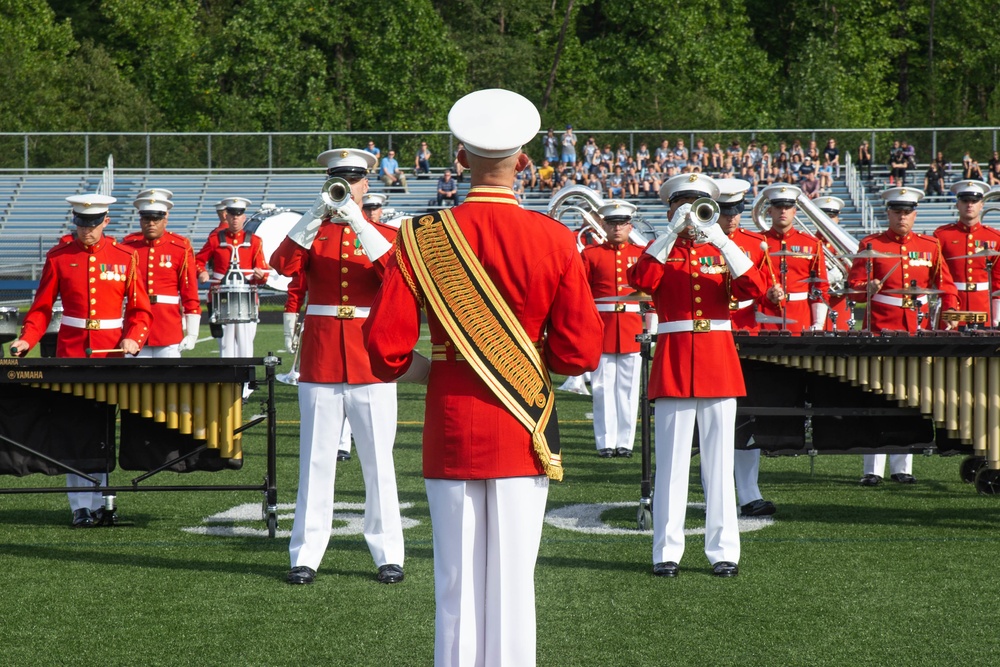The image depicts a distinguished marching band, likely from the marines, performing on a football field. The band members are attired in striking red jackets adorned with golden buttons and badges, paired with crisp white slacks and flat white hats. The uniform of the man leading the band is notably distinguished by a gray sash draped across his chest and shoulders, indicating a position of importance or royalty. In front of the conductor, trumpet players are prominently featured, followed by xylophone players and other percussionists, including a marimba and drums positioned to the left, with tuba players and cymbals to the right. The backdrop includes a lush, green landscape with trees, and the football field's stands are filled with spectators, notably children, observing the band's performance.